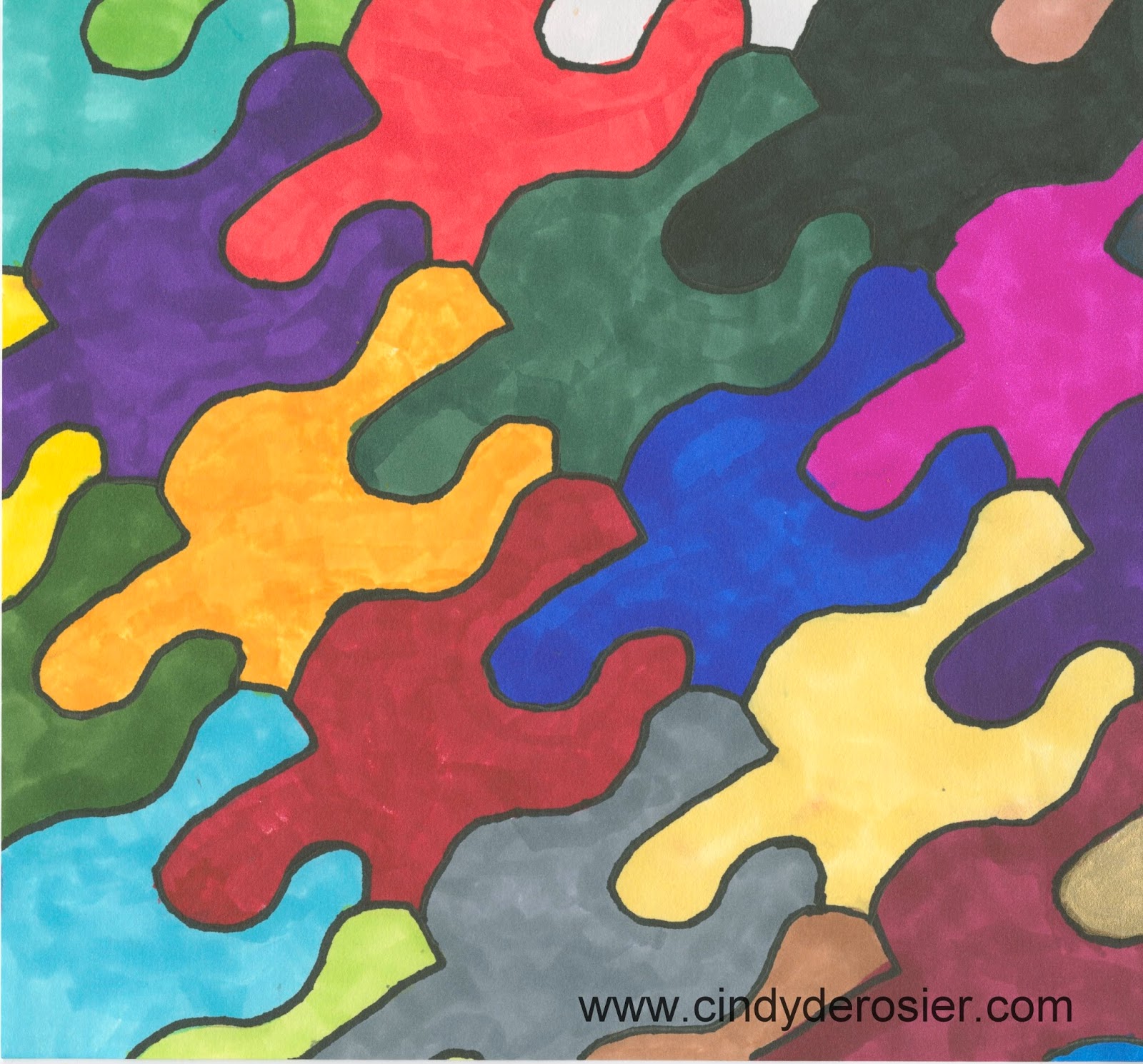This image appears to be a color photograph of a marker illustration showcasing a series of identical puzzle piece-like shapes, all interconnected and arranged in rows and diagonals. Each piece is outlined in black marker and filled in with various vibrant colors, including yellow, red, blue, green, purple, orange, and more. The repetitive patterns suggest that stencils were used to maintain the uniform shape of each piece. The arrangement of shapes gives a dynamic impression, with each row pointing diagonally to the right, creating an interlocking, overlapping effect. The artwork, which can be seen as a mural or wall art, might symbolize unity and connectivity. At the bottom right corner of the image is the text "www.cindyderosier.com," marking the creator's website. The vivid colors and structured layout make this piece visually captivating, resembling a harmonious blend of art and design.